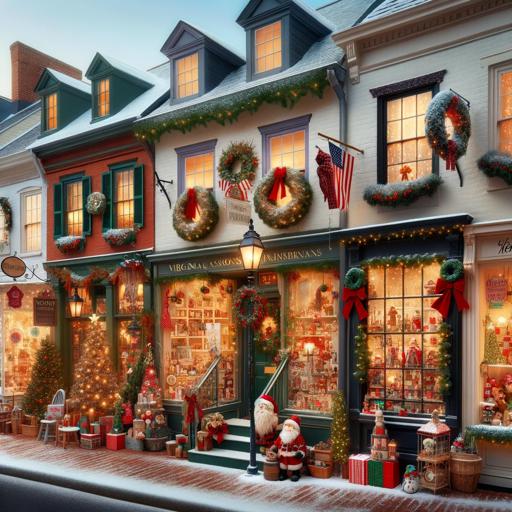The image depicts a festive storefront that is part of an enchanting row of buildings, reminiscent of New England architecture. The two-story buildings have dormer windows on the rooftops, with the second-floor windows adorned with Christmas wreaths, red ribbons in the flower boxes, and some waving American flags. The storefront itself is highly decorated for the holiday season, with a green exterior and wide picture windows that offer a peek into a wonderland of Christmas decorations.

The center store, bursting with holiday cheer, is filled with an array of Christmas trees, Santa statues, gift boxes, and toys. Outside, a line of Christmas trees adorned with glowing stars and twinkling lights stands next to the front stoop, where little Santa figurines add to the festive atmosphere. The green steps leading up to the door are covered with a light layer of snow, and the sidewalk in front is similarly dusted. The windows of the store are trimmed with lights, wreaths, and red bows, showcasing a variety of Christmas items both inside and out, making it a true winter wonderland.

Overall, the image captures a beautifully decorated city street celebrating Christmas, complete with snow-covered sidewalks and a storefront that looks almost magical, whether it's a heavily photoshopped photo or an incredibly realistic painting.